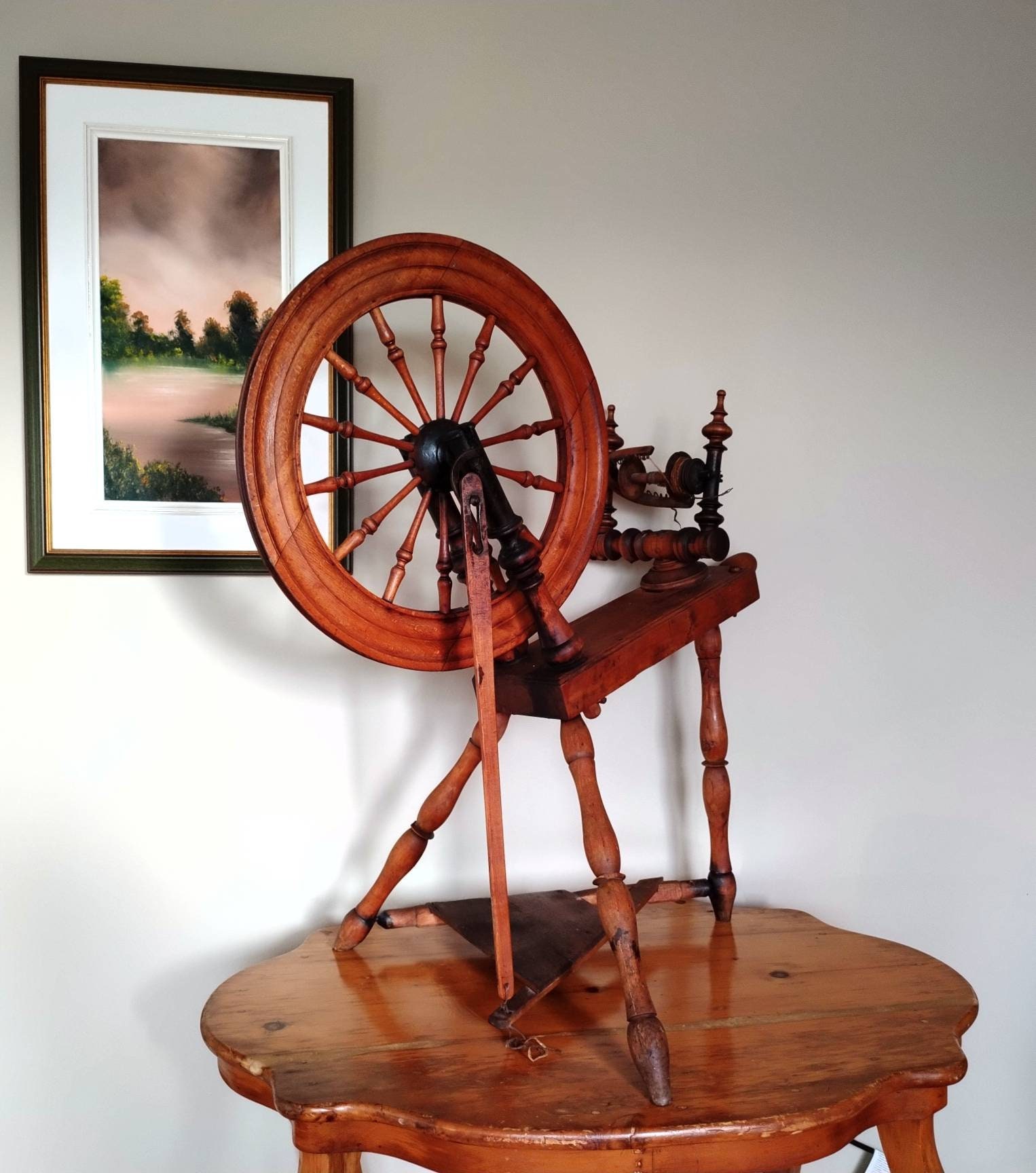The image depicts a vintage spinning wheel, meticulously positioned in the center of a small brown table. The spinning wheel, primarily walnut brown, features some black elements, possibly painted or metallic, mainly around the center. It stands on three sturdy legs, with a minor support connected to the wheel. The design resembles an old ship's steering wheel, complete with a pedal and a stick attached to it. Two spools are visible, designed to hold thread or wool, which is processed into yarn as the pedal is operated. This intricate apparatus is set against a white wall, with a framed painting of a lake with trees hanging to the top left. The colors prominent in the image include shades of walnut brown, gray, black, yellowish gold, green, and white, creating a warm, earthy ambiance in what appears to be a cozy home setting.